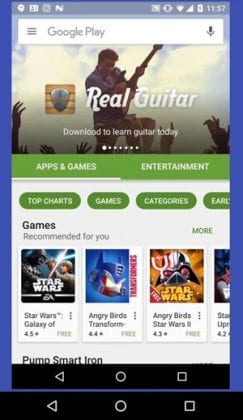This image is a detailed screenshot of the Google Play Store interface. At the very top, there are four icons on the upper left. On the upper right, there are several icons including the Wi-Fi icon, cell phone reception icon, two additional icons, and the battery icon. The time displayed is 11:57. Below this top section, there is a Google Play search bar. Behind the search bar, there is an advertisement banner featuring an image of a person playing the guitar, with the text "RailGuitar" and "Download to learn guitar today." Below the ad, a green navigation bar indicates different sections of the store, with "Apps & Games" selected. Further down, there are four tab options: "Top Charts," "Games," "Categories," and a partially visible tab that starts with "Early." Following these tabs, the screenshot displays thumbnails of three game apps.